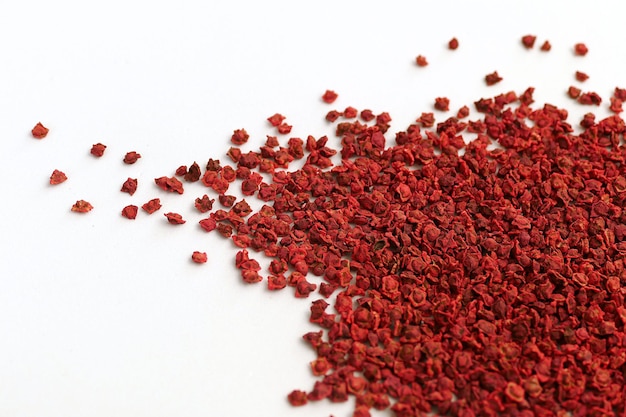In this image, set against a white background, there is a scattered pile of red, pellet-like objects, concentrated primarily in the bottom right quarter. The small pieces vary in shape, some being roundish while others are elongated or irregular, with some appearing double-layered. They exhibit shades ranging from deep blood red to occasional hints of brown. The objects, possibly resembling potpourri, tiny gravel, or even aquarium rocks, spread out sparsely from the main concentration towards the middle and left sides of the image, creating a dispersed pattern. The overall effect is a dynamic distribution of these unknown red elements across the white backdrop.